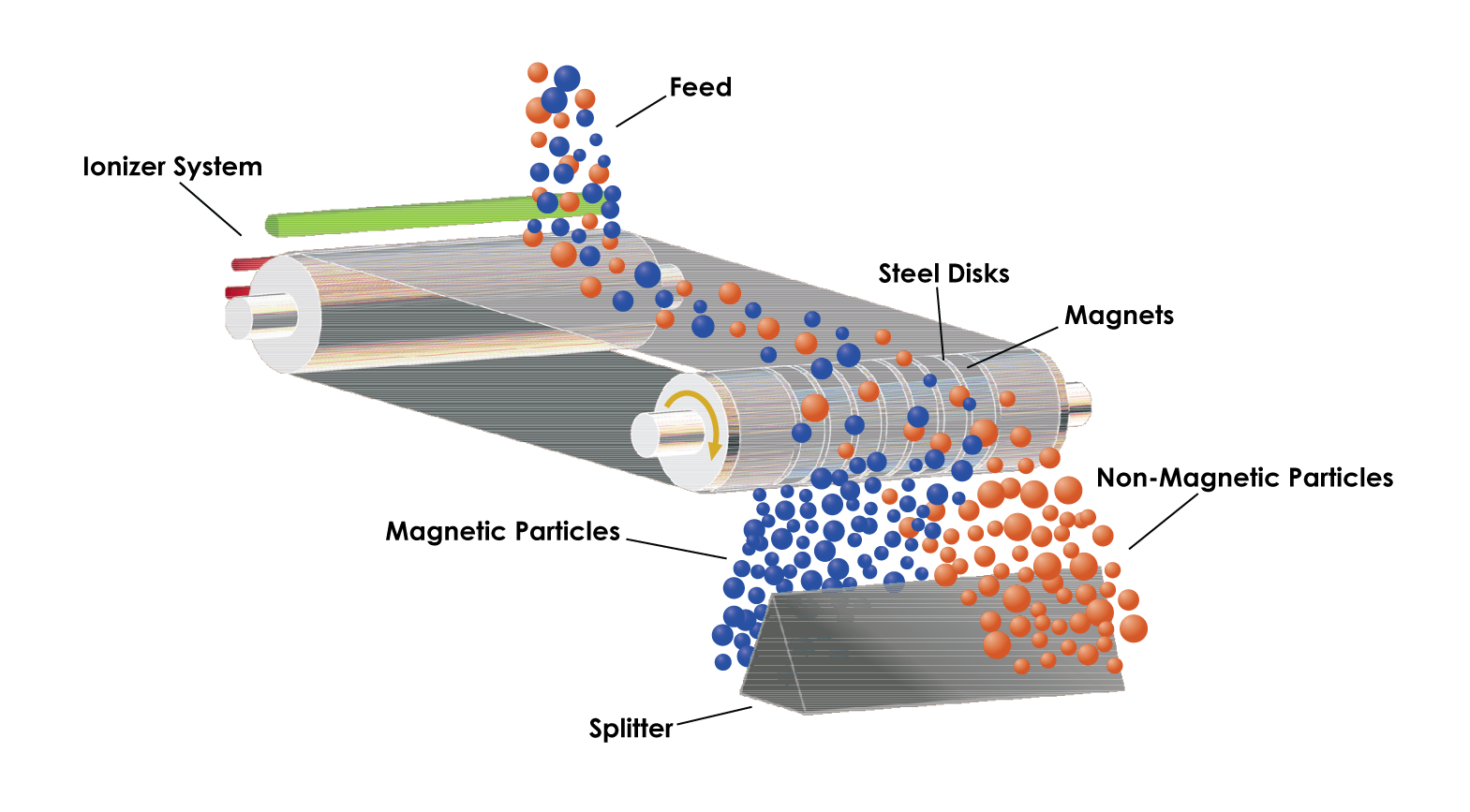This is a detailed horizontal drawing of an ionizer system featuring a conveyor belt designed for the separation of magnetic and non-magnetic particles. The belt, equipped with green, silver, and gray rollers, directs blue and orange particles—representing magnetic and non-magnetic materials, respectively—down its length. As the particles travel on the belt, they are sorted as they approach a splitter. The blue, magnetic particles are pulled towards an area with steel discs and magnets located on one side, causing them to fall to the back side of the splitter. Conversely, the orange, non-magnetic particles, unaffected by the magnets, continue on their path and are directed to the other side of the splitter. This setup is engineered to effectively divide ferrous materials from non-ferrous ones along the conveyor belt system.